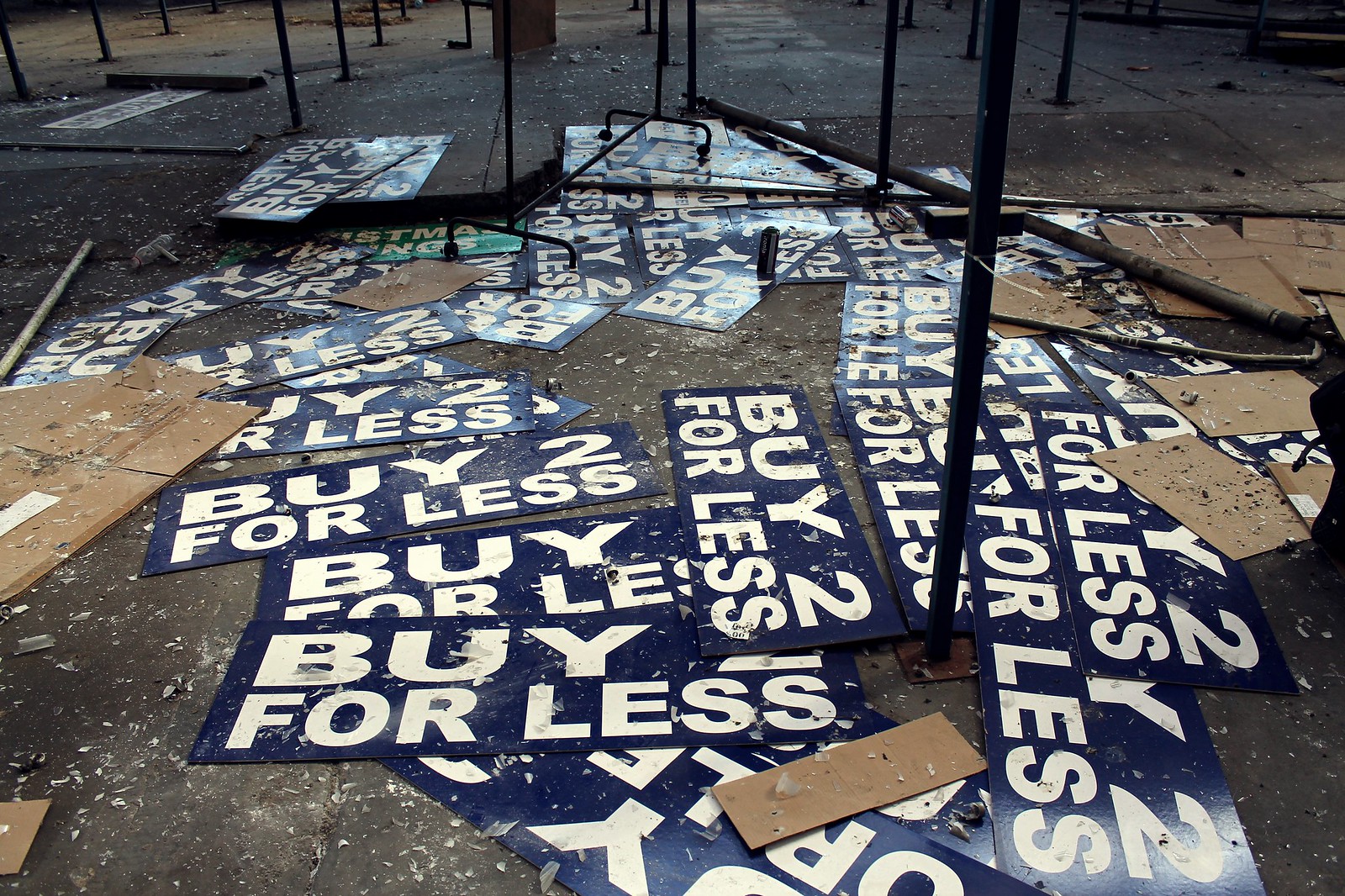The image depicts an interior of what appears to be an abandoned retail space or warehouse, characterized by a barren, dusty concrete floor littered with debris. Scattered haphazardly across the ground are numerous blue rectangular signs with bold white text reading "Buy Two for Less," some of which are flipped upside down, revealing their brown backs. Among these are other scattered materials, including pieces of cardboard. In the background, a black rolling clothes rack and several black metal poles extend upwards, likely toward the ceiling, although this part of the image is not fully visible. Additionally, a diagonal pole lies across the floor in the upper right corner, and a possible support beam for the building is visible in the center top area of the image. The overall atmosphere conveys a sense of neglect and disarray.